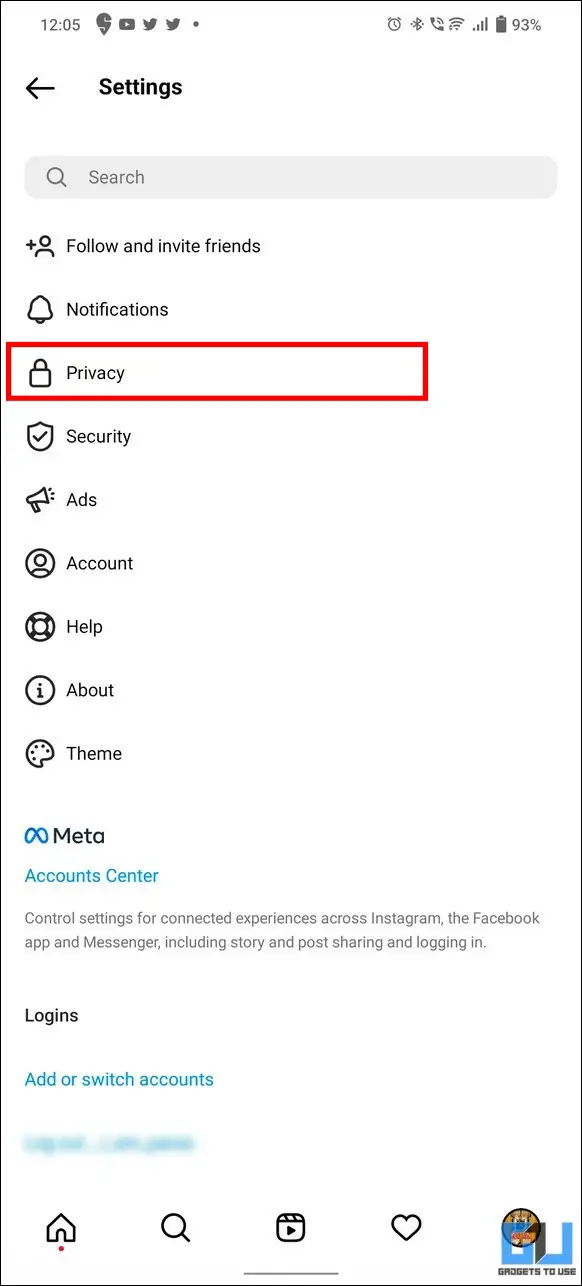The image showcases a settings screen on a mobile device. In the bottom right corner, there is a blue and black logo that reads "Gadgets to Use" with the initials GU. The top-left corner displays the time as 12:05. Adjacent to this are various icons including a YouTube play button, Twitter icons, and in the top-right corner, icons for alarm clock, Bluetooth, phone, Wi-Fi, data signal, and a battery life indicator at 93%. 

Below the status bar, a black back button labeled "Settings" is present with a gray search bar beneath it. The screen lists several options: Follow and Invite Friends, Notifications, Privacy, Security, Ads, Account, Help, About, and Theme.

Further down, the Meta logo (an infinity symbol) appears next to the word "Meta," accompanied by the text "Accounts Center," detailing control settings for the interconnected experience across Instagram, Facebook app, and Messenger—including story and post sharing, and logging in. There's a section for "Logins," including a blue button labeled "Add or Switch Accounts."

At the bottom of the screen, a navigation bar displays a home icon, a magnifying glass, a play button, and a heart icon.